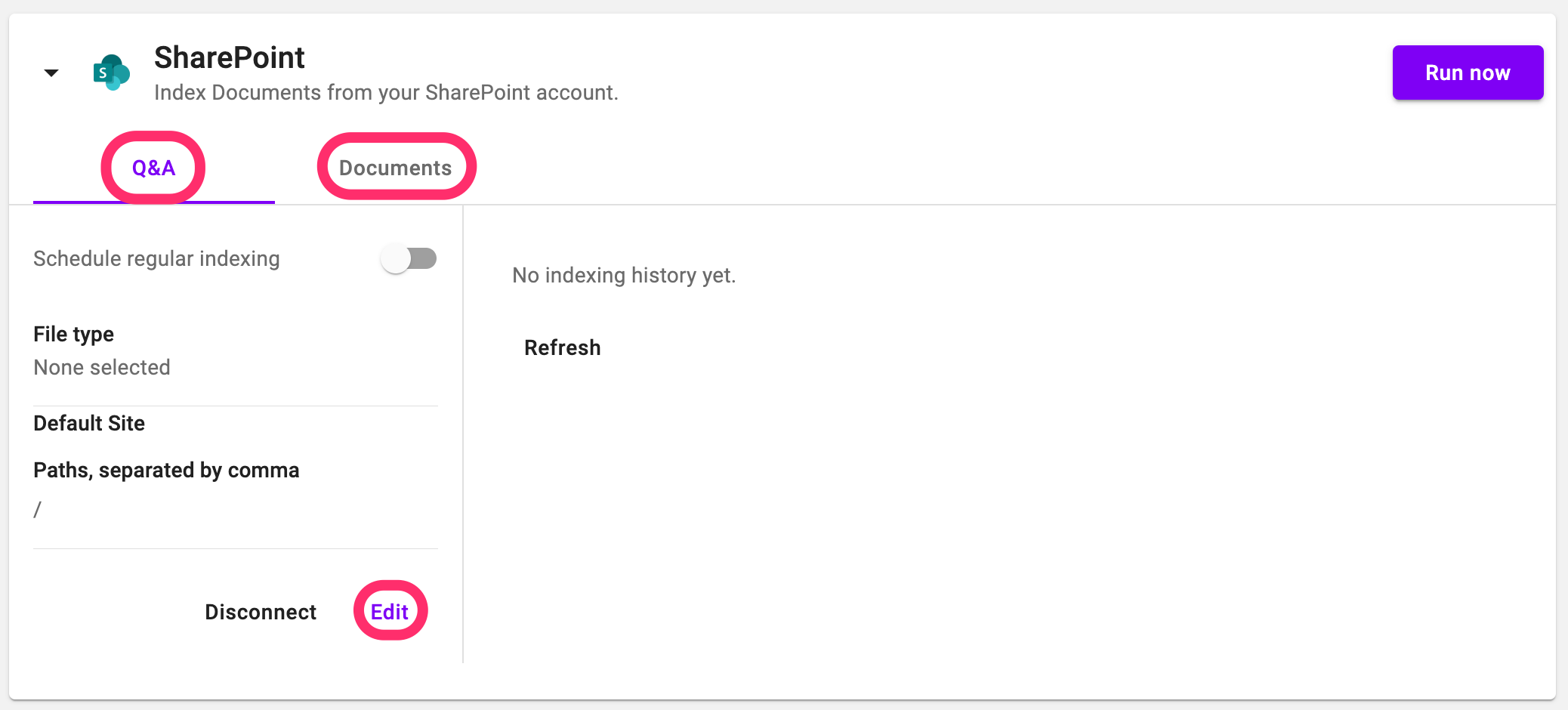This image captures the user interface of a SharePoint backup folder, displayed in landscape orientation with approximately twice the width compared to its height. The screen is bordered by a prominent shadow, set against a pristine white background, which accentuates the content within.

At the top of the screen, there is a drop-down caret adjacent to the SharePoint icon, which is distinguished by its green color and design featuring an "S" accompanied by a collection of circles and a square. Following the icon, the title "SharePoint" appears in bold black font, accompanied by the subtitle "Indexed documents from your SharePoint account."

To the right of the SharePoint title, a prominently placed purple rectangular button with rounded edges, containing white text, invites users to "Run Now."

Below this header section, there are two tabs: "Q&A" and "Documents." The "Q&A" tab is highlighted in purple with an underline, indicating it is currently active. Both tabs are encircled— "Q&A" in a red circle and "Documents" in a red oval.

Underneath these tabs, the text "Schedule regular indexing" appears, along with a toggle switch that is currently set to the "off" position. Further down, users are presented with input fields labeled "File type," "Default site," "Paths separated by comma," and buttons for "Disconnect" on the left in black and "Edit" on the right in purple, with the "Edit" button encircled in red.

A gray vertical divider splits the screen, with the right half displaying the message "No indexing history yet." Nearby, there is a refresh button, enabling users to update the displayed information.

Overall, the image serves as a detailed visual guide for setting up and managing indexing and backup operations within a SharePoint site.